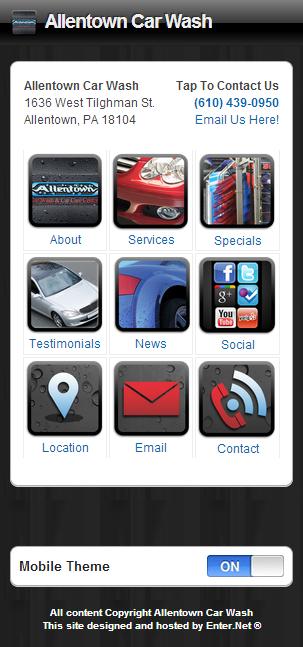The image appears to be a vertically aligned rectangle, akin to a smartphone screen, likely a screenshot of an app interface for Allentown Car Wash. The top of the image features a black and grey frame with white letters that read "Allentown Car Wash." Below this is a white rectangular background displaying the business’s address in black font: "Allentown Car Wash, 1636 West Tilghman Street, Allentown, Pennsylvania, 18104." It also includes the clickable prompts "tap to contact us" alongside a blue phone number "610-439-0950" and a directive to "email us here!" 

The middle section consists of nine square icons arranged in a grid, each representing different sections and functionalities. The icons include:
- About: Featuring info about the business.
- Services: Depicting a car's headlight.
- Specials: Illustrated by a toolbox.
- Testimonials: Showing a car driving down the road.
- News: Highlighted by a car's fender.
- Social: Displaying social media icons such as YouTube and Facebook.
- Location: Represented by a map location arrow.
- Email: Indicating where emails can be sent.
- Contact: A phone icon for direct calling.

Each icon is accompanied by corresponding labels under them. 

At the bottom of the image, there is a white bar with the text "mobile theme" in small white print and an "on" button set against a blue background. Below this, there is a note stating "All Content Copyright Allentown Car Wash" along with a mention that the site is "designed and hosted by Internet," followed by the trademarked address "enter.net™".